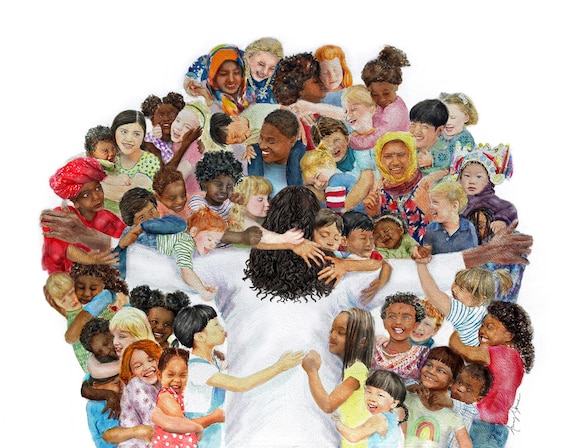The digital illustration depicts a diverse group of people, predominantly children from various ethnic backgrounds and nationalities, gathered around a figure who appears to be Jesus. Jesus, seen from behind, has long, curly, dark brown hair that extends past his shoulders, and he is wearing a long white robe. His arms are extended outward, welcoming the children who are encircling him joyfully. The children and a few adults are shown in an array of different clothing styles, reflecting their varied cultures and religions—some are wearing hijabs, turbans, and traditional attire from various regions. The scene is vibrantly inclusive, showcasing individuals of all ages, skin tones, hair textures, and clothing colors. Everyone is smiling, expressing happiness and unity as they reach out and hug one another, forming a harmonious and interconnected circle around Jesus.